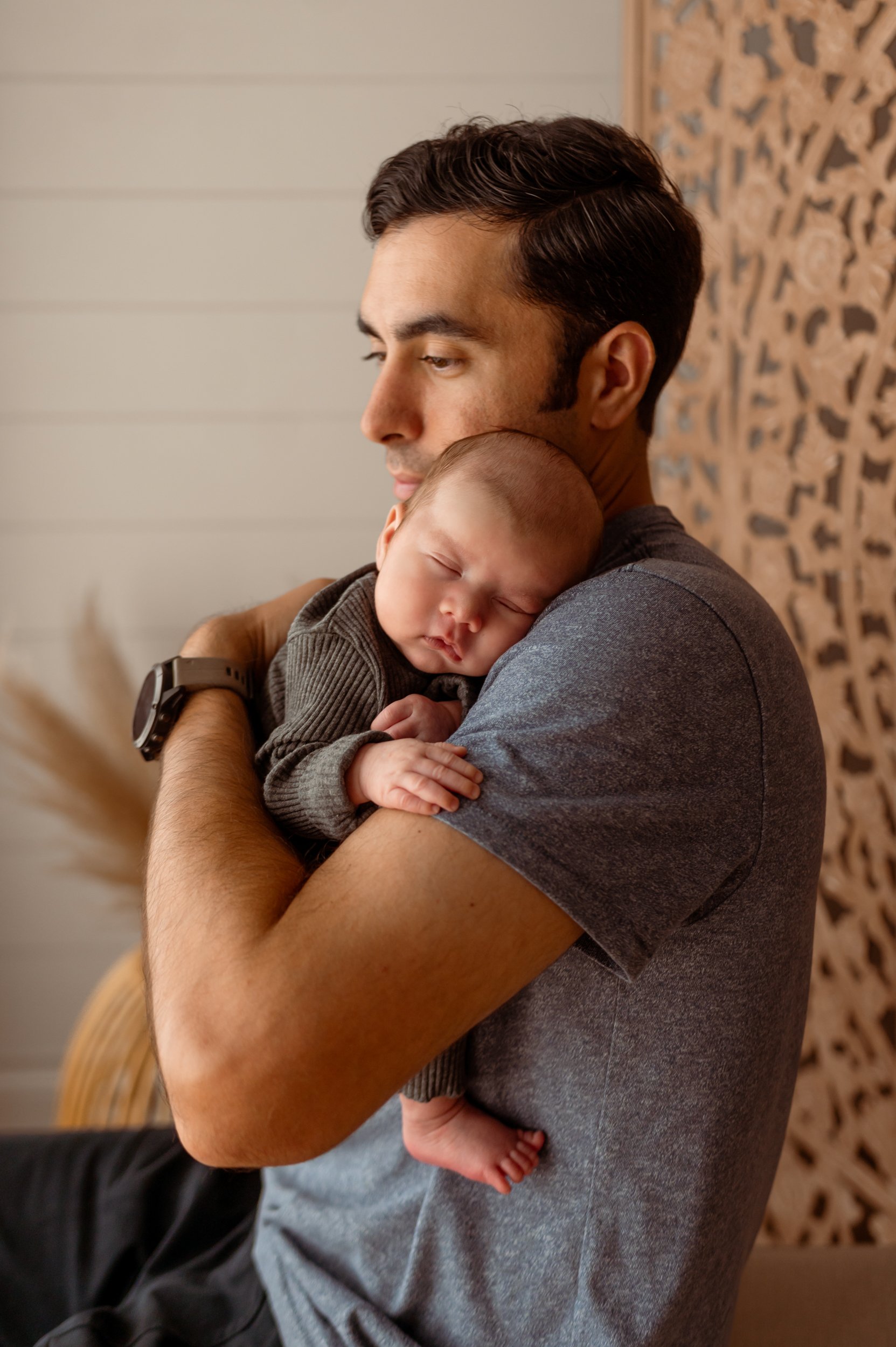This intimate close-up photograph captures a young father tenderly cradling his sleeping infant son against his shoulder. The father, who has brown eyes and brown hair, wears a blue-gray jersey-style t-shirt and black pants. His expression is pensive, and he gazes slightly downward and to the side while holding his son securely. The large sports watch with a brown leather band on his left wrist is visible as the baby's tiny hand gently touches his arm. The baby, dressed in a simple gray sweater and without shoes, appears content and deeply asleep, nestling comfortably into his father's shoulder. The background features a blend of white wooden panels and an intricate, beige Chinese-style screen, adding an element of elegance to the scene. Additionally, a lovely beige plant in a vase is subtly visible, contributing to the serene ambiance of the setting.